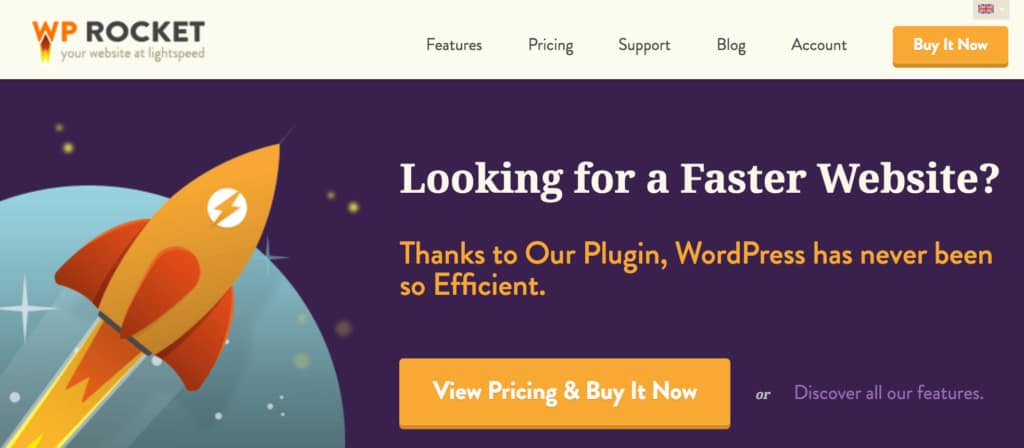This image is a screenshot from a website featuring the WP Rocket plugin. The top section prominently displays "WP Rocket" alongside the tagline "Your Website at Light Speed." An illustrative rocket streaks under the letter "W." The navigation menu includes tabs for Features, Pricing, Support, Blog, and Account, with a vibrant orange "Buy It Now" button featuring white text.

The main visual element beneath the navigation is an eye-catching rocket on the left, set against a deep purple background with subtle orange highlights that simulate outer space. Above the rocket, white text poses the question, "Looking for a faster website?" Below this, in bold orange text, it claims, "Thanks to our plugin, WordPress has never been so efficient."

At the bottom, the image features an orange box with white text that reads "View Pricing and Buy It Now." Beside this box, purple text offers an additional option: "or discover all of our features."